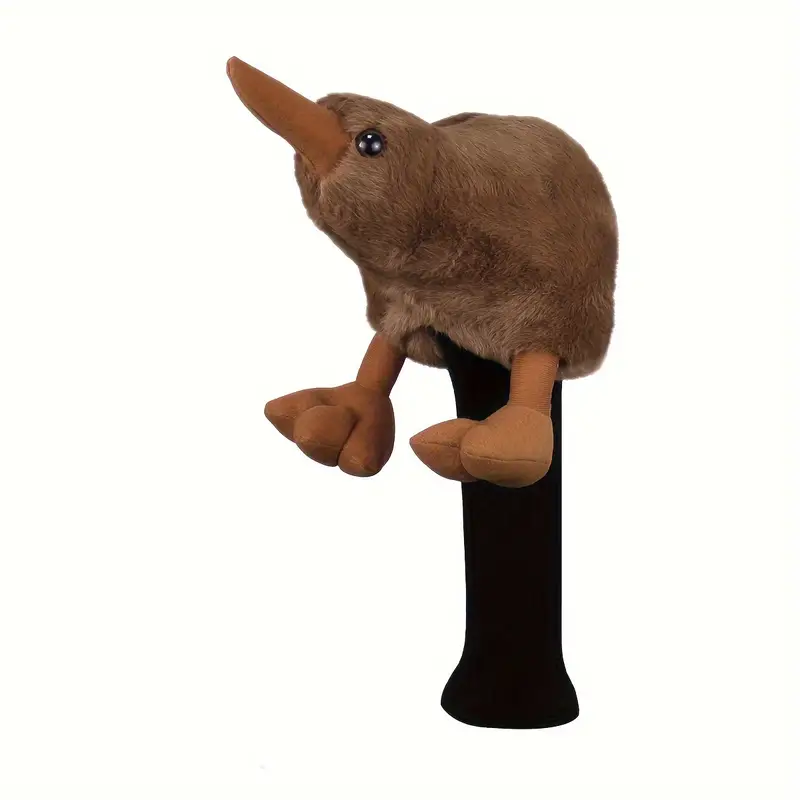In the image, against a white background, a toy duck with a furry appearance is displayed atop a dark brown to black stick. This stick, which serves as a display holder, rises up from the bottom and firmly supports the stuffed animal. The plush duck exhibits a mixture of light brown, dark brown, and standard brown furs, giving it a rich and textured look. The duck, characterized by a very dark orange beak and dark black beady eyes that reflect a small glare, is positioned to gaze upward towards the left-hand upper corner. Its two deep orange legs, each ending in three well-defined toes, protrude from the base of its round, ball-like body. A subtle crease can be seen on its back. Despite varying descriptions, the consensus is that this is a uniquely posed toy duck, possibly even a hand puppet, accentuated by its articulated features and supported prominently by the sleek, dark stick.